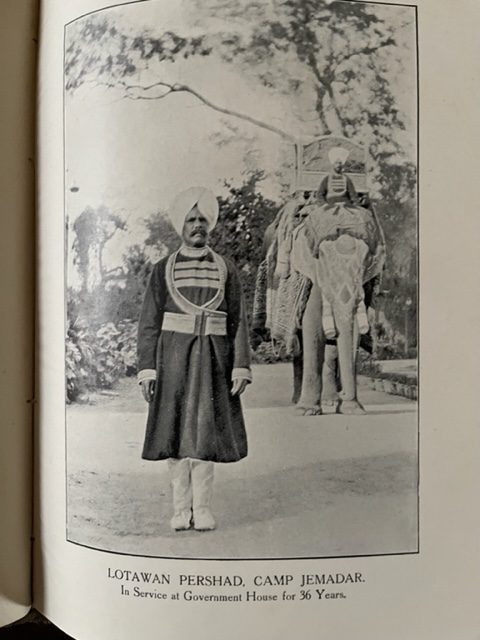The photograph, taken from the right-hand page of a book, is primarily in black and white or grayscale, emphasizing an old and historic feel. To the left, one can see the crease at the book's spine. Central to the photograph is Latawan Prashad Kamp Jemadar, noted for his 36 years of service at Government House, as denoted by the caption beneath the image. He stands in a long, decorative coat extending to just below his knees, adorned with stripes across his chest, and sports a white turban and mustache. His ensemble includes white pants and white shoes. Behind Jemadar is a grandly adorned elephant, bedecked with blankets and artwork on its face. Seated atop the elephant is another man, dressed similarly, riding in a large chair or cabinet on the elephant's back. The scene is set on a dirt road, flanked by trees and bushes, adding a natural backdrop to this intriguing historical snapshot.